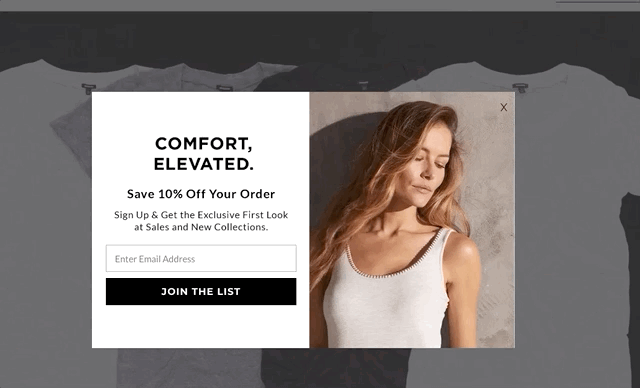The image displays a screenshot featuring a promotional pop-up over a stylized background. The backdrop is predominantly black with a subtle gray pattern, resembling the outlines of t-shirts. Dominating the foreground is a square pop-up window, partially cut off on the left side, with a clean white background and bold black text. The text reads, "Comfort Elevated. Save 10% off your order. Sign up and get the exclusive first look at sales and new collections." Directly beneath this message is a plain white email address input field, labeled with engraved text, "Enter email address." Below the input field, a prominent black button with white lettering invites users to "Join the List."

To the right of the pop-up is a photograph of a Caucasian woman with light brown, almost blonde hair, leaning against a wall. Her eyes are closed, and she is facing slightly to the viewer's right. She is wearing a white tank top and appears to be bathed in sunlight. An "X" in the upper right-hand corner of the pop-up allows users to close the window. This succinctly describes the content of the screenshot.